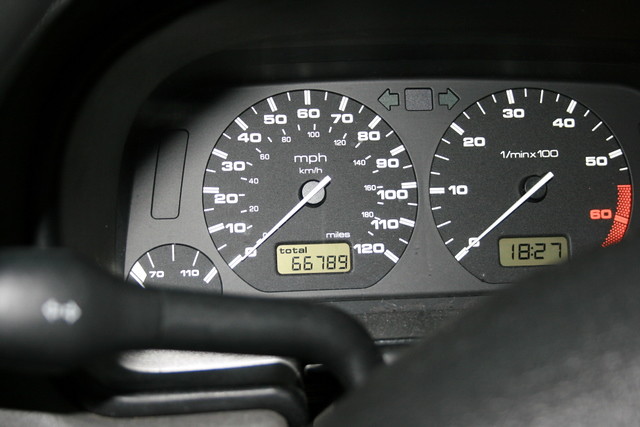The photo showcases a close-up view of a vehicle's dashboard, featuring both digital and analog displays. Prominently, the digital odometer reads 66,789 miles. The speedometer, marked with both miles per hour and kilometers per hour, currently indicates 0 mph but extends up to 120 mph. Adjacent to the speedometer is a temperature gauge designed to alert the driver if the vehicle overheats.

Also visible are indicator lights for turn signals, with both left and right signals clearly marked, and dual signals likely used for hazard lights. The RPM gauge is at 0, and the digital clock displays the time as 18:27, or 6:27 PM in military time. The dashboard itself is black, and a portion of the steering wheel is visible, along with the turn signal lever peeking out from beneath the dashboard.